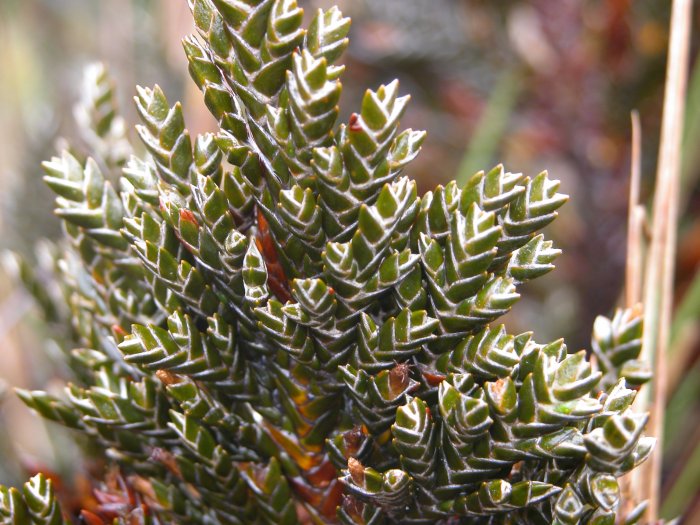The image features a close-up of a unique, cactus-like succulent plant as the central focus, captured with a bokeh effect that blurs the background. The plant exhibits thick, spiny, and stubbier leaves reminiscent of both cacti and succulents, and is characterized by a green hue with white edges. The short, pointy leaves grow from whiny twigs branching off a main stem, which is deep red and light orange in color towards the base. In the lower-right corner of the image, there’s a hint of a vertical beige shaft, perhaps a straw or some part of the plant itself. The blurred background features indistinct green and red coloring, enhancing the central plant's striking appearance.